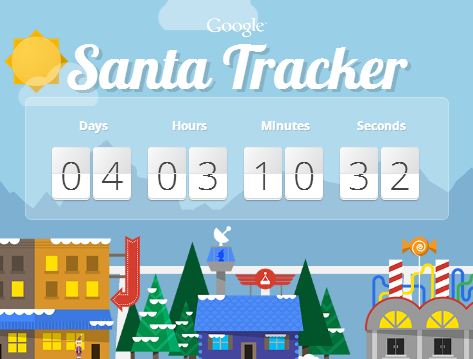In this image of Google's Santa Tracker, we see a vibrant, cartoon-style interface against a light blue background representing the sky. At the top of the square box, "Google" is prominently displayed in white, with "Santa Tracker" written below it. To the left, a cheerful yellow sun adds to the festive atmosphere.

The scene is populated with colorful, cartoon-drawn buildings adorned with snow and festive decorations. One building features an array of candy canes and candies, adding a whimsical touch to the landscape. Snow blankets the rooftops and the surrounding trees, enhancing the wintery feel.

A large red arrow, resembling a directional sign, points towards the buildings, drawing attention to the countdown timer below. It reads: "4 days, 3 hours, 1 minute, and 32 seconds until Santa arrives," building excitement for the holiday event.

In the bottom left of the image, there's a small, purple house-like building with a blue roof, standing out amidst the snowy, candy-filled scene. The overall composition is playful and inviting, perfectly capturing the spirit of anticipation for Santa’s arrival.